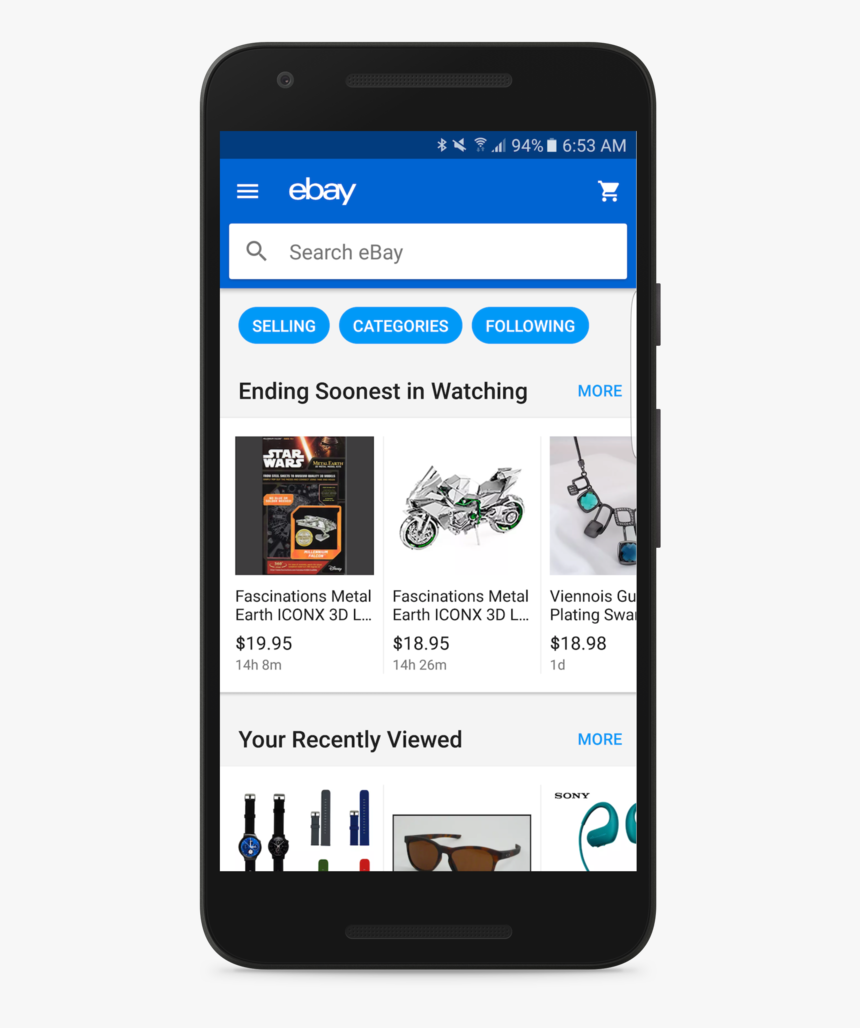A black iPhone-style cell phone is showcased against a gray background. The phone, with an entirely black exterior including the top, bottom, sides, and buttons, is displayed with its screen facing the viewer, revealing a website.

At the top of the screen, a status bar displays icons from left to right: Bluetooth, a muted speaker (with a line through it), Wi-Fi signal, cell signal, a battery indicator showing 94%, and the time at 6:53 A.M. Below the status bar, a lighter blue banner features three horizontal white lines on the left side, the word "eBay" in the center, and a shopping cart icon on the right.

Immediately below this banner, a search bar reads "search eBay" with a magnifying glass icon. The next section, set against a light gray background, presents three options: "selling," "categories," and "following." Underneath, the page lists "ending soonest," "watching," and a "more" button in a blue font.

The main content section displays a series of items: Starting with "Fascinations, Middle Earth, Iconics, 3D, $19.95," followed by "Fascinations, Middle Earth, Iconics, 3D, $18.95," and another heading "Vienois" which is partially cut off, showing "GU." Another listing reads: "Splitting, S-W-A," also cut off, priced at $18.98. The last visible text hints at a "recently viewed" section that is partially obscured.